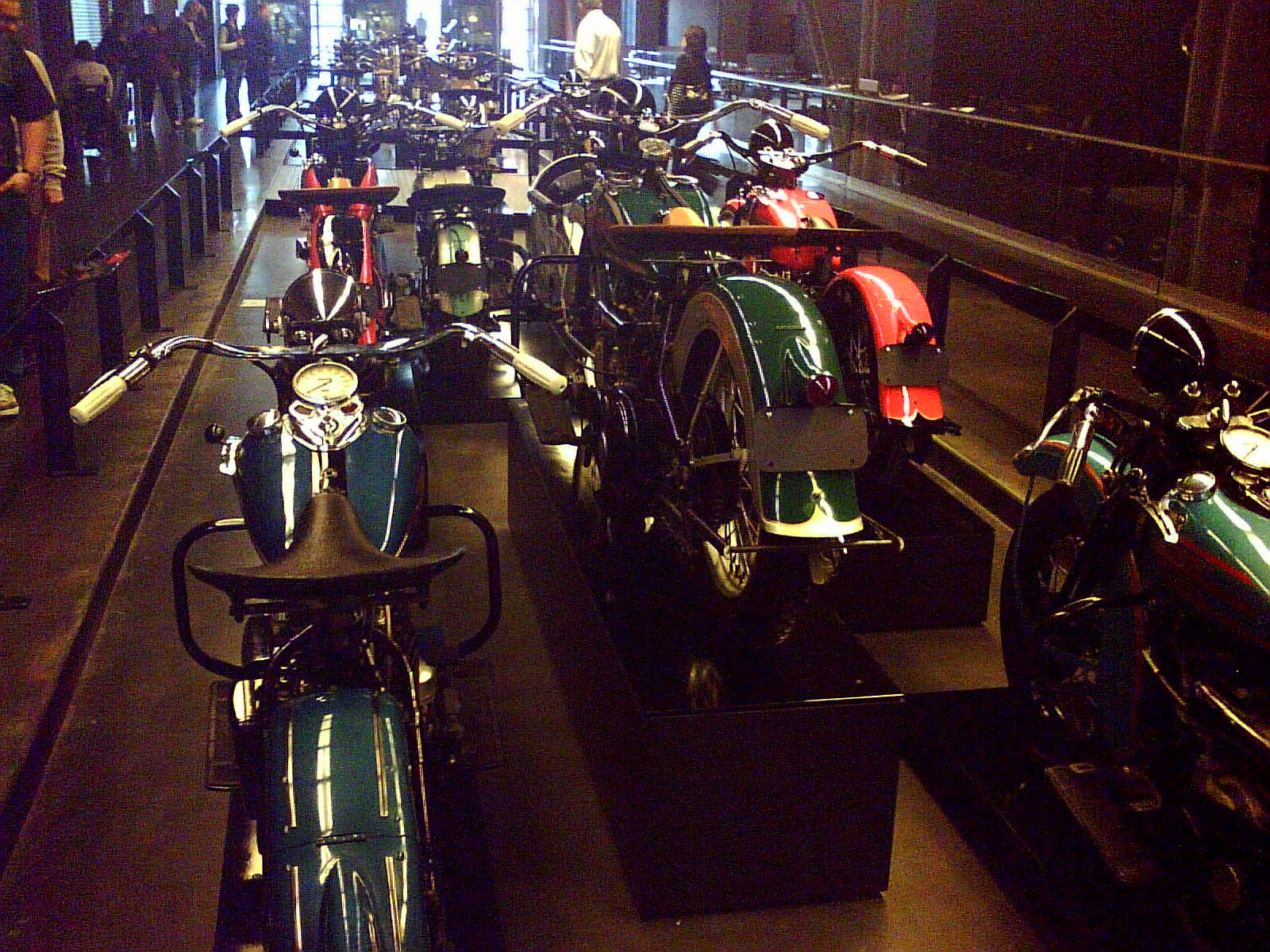This image taken inside a museum showcases a stunning display of vintage motorcycles, all impeccably restored and gleaming in various colors including blue, green, red, and white. The motorcycles, numbering at least seven in the visible foreground with possibly more extending into the background, are set on rectangular wooden pedestals, positioned within a dedicated viewing area. The exhibit is surrounded by wooden railings and bordered by glass barriers on both the left and right sides. Visitors, including a man in a black t-shirt and a person in a wheelchair, are seen standing on the left side, captivated by the collection. The right side of the image reveals another barrier and reflective windows. The room itself features many wooden accents, and natural light or enhanced lighting illuminates the space as it extends further into the distance, highlighting the pristine condition of these antique motorcycles.